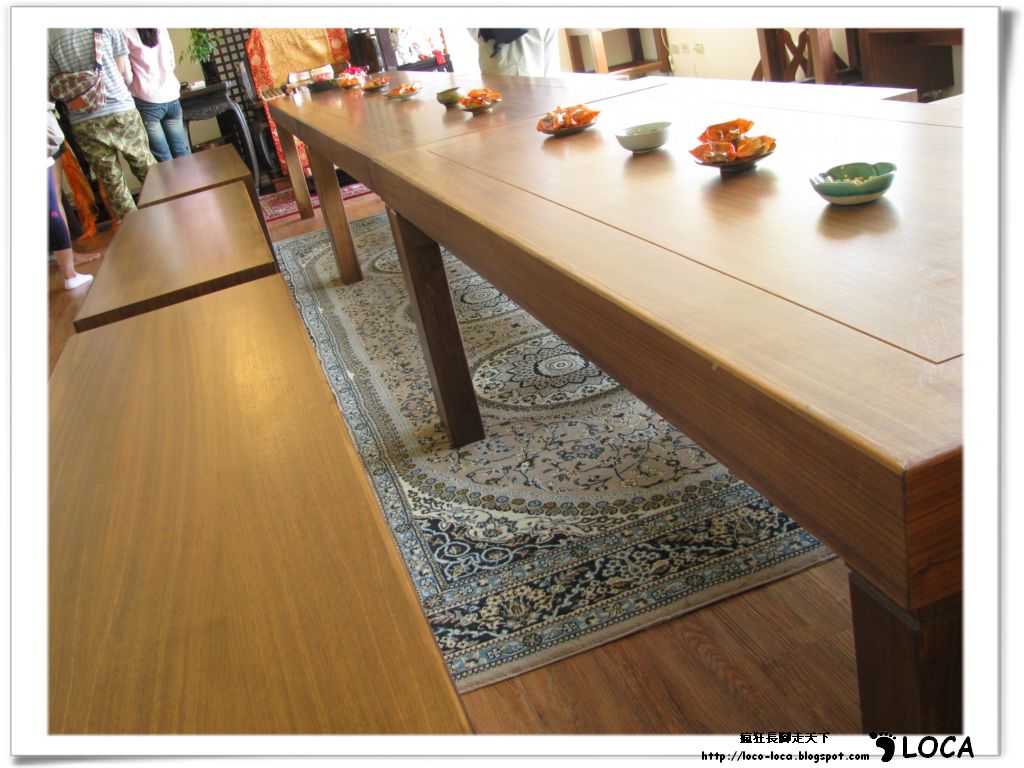This photograph, likely taken inside a restaurant, captures a long wooden table adorned with a repeating pattern of ceramic arrangements, consisting of small greenish-blue bowls, orange items set on small plates, and white bowls. This sequence extends down the length of the table. Beneath the table lies a colorful oriental rug, situated over a wooden floor. Adjacent to the table are three long wooden benches. In the distant background, near another table or desk, several people can be seen, including a man in green military-style pants with a black and white striped shirt and carrying a red and white sling bag, and a woman in a pink shirt paired with blue jeans. Visible text at the bottom right of the image reads "http://loco-loco.blogspot.com" alongside an image of a footprint and the word "LOCA" in bold.